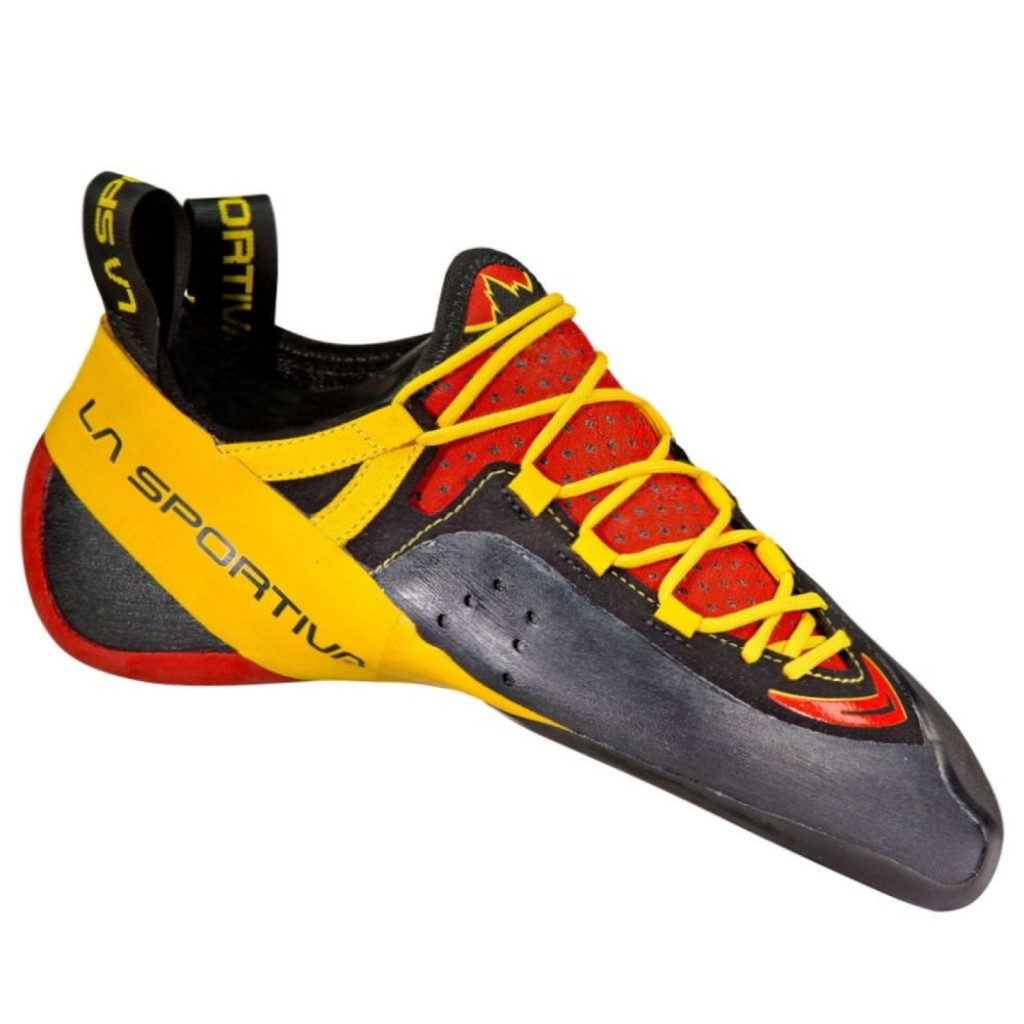This close-up image depicts a uniquely designed athletic shoe by LA Sportiva, incorporating colors of yellow, red, and black. The shoe exhibits an unconventional shape with a pointed, rubbery black nose and a slightly bent tip, suggesting it fits snugly on the foot. It features yellow laces that serve as slip-on straps rather than traditional laces. Red accents outline the heel and tongue, complementing a triangular yellow band on the side emblazoned with the brand name. The backside shows strap-like laces with similar branding, aiding in slipping the shoe on. The overall footwear design is sleek, smooth, and lacks visible tread on the sole, with a blend of functional aesthetics and athletic precision.